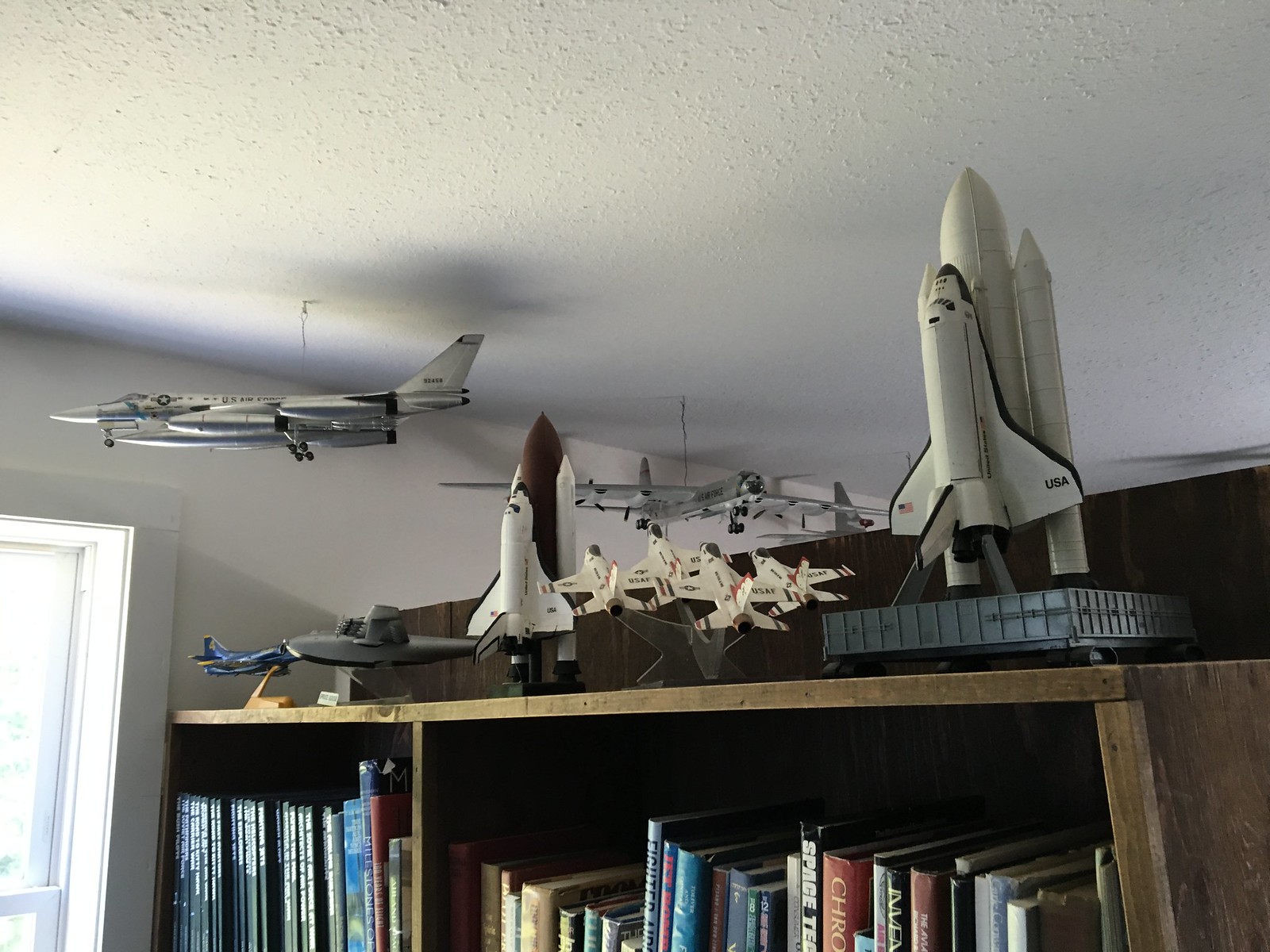This image showcases the top of a wooden bookshelf, adorned with an intricate collection of model spacecraft and aircraft. The top shelf is lined with books, whose upper halves are visible, filling the two sections of the shelf completely. Atop the shelf stands an elaborate array of space shuttle models, noteworthy are the Challenger-type space shuttles poised as though ready for launch, complete with towering central booster rockets in dark brown and flanked by smaller white rockets on either side. Additionally, a striking blue jet with a light blue top and dark blue wings can be seen, its nose pointed left. Adjacent to it, a sleek gray submarine model faces the same direction. Among these is another space shuttle model, set on a substantial black base, its pristine white body accentuated with black details around the wing tips, also aimed towards the ceiling. Nearby, another formation shows four white fighter jets, each marked with black lettering, angled upwards and to the left. 

Hanging from the white ceiling are two more impressive aircraft models: a larger passenger plane and a silver jet, both suspended by wires. The jet in the foreground has its nose pointed left, while another jet in the background aims towards the camera and slightly to the right. On the left side of the image, the border of a window peeks in, casting natural light onto the scene and framed with a white border. This eclectic collection hints at a dedicated space enthusiast, with one of the visible book titles bearing the word "space," indicating a likely theme among the amassed literature.